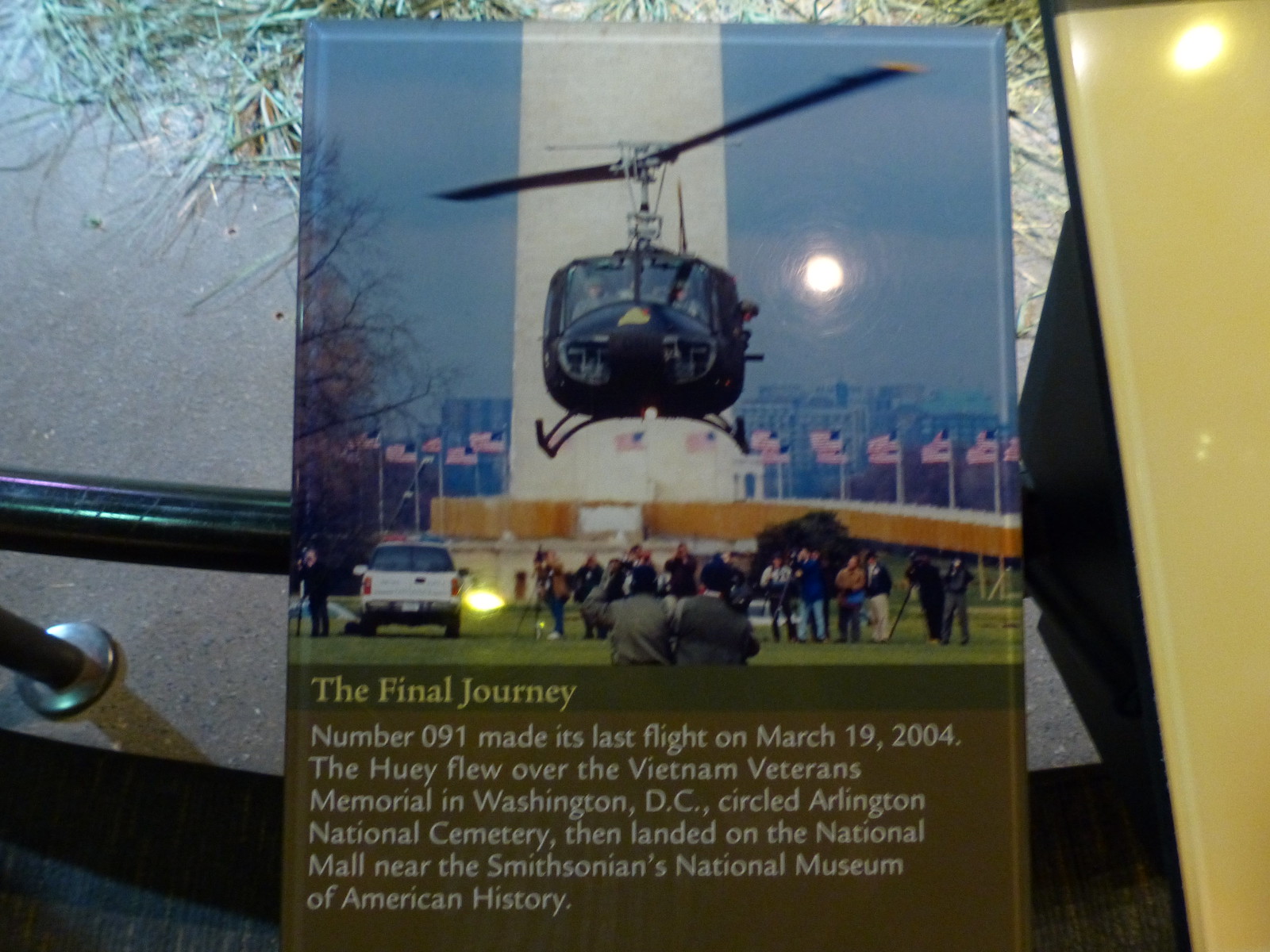This detailed image captures a plaque dedicated to the final flight of the famous helicopter, Huey, which is immortalized for its historical significance. The plaque features a photograph of the Huey landing on the National Mall near the Washington Monument, surrounded by reporters, cameras, and many people standing on the grass, encircled by American flags. The scene also includes a white truck parked nearby. The text on the plaque, in white font on a green background, prominently describes "The Final Journey" of Huey, number 091. It meticulously details how this iconic helicopter made its last flight on March 19, 2004, flying over the Vietnam Veterans Memorial, circling Arlington National Cemetery, and concluding its journey near the Smithsonian's National Museum of American History. The left side of the plaque shows a pole, while the right side partially reveals another framed photograph with a noticeable yellow frame.